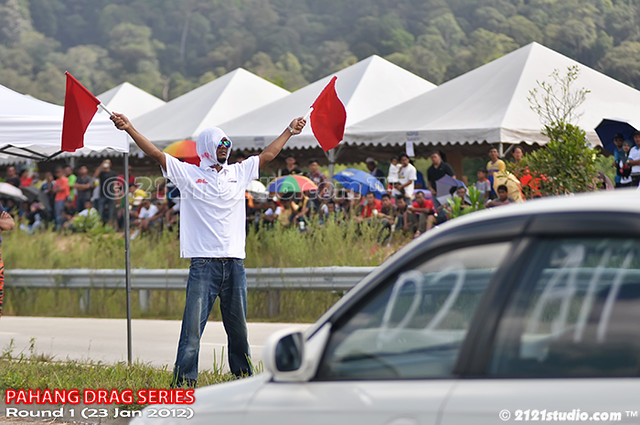This outdoor photograph, taken during the daytime at a drag strip event, captures the high-energy atmosphere of the Pahang Drag Series Round 1 held from January 21-23, 2012. The image is rectangular and features a dynamic scene with a central figure poised to signal the start of a race. This man, dressed in a white shirt, a hood, and blue jeans, stands in an 'X' position holding two red flags, marking the beginning of a race. He is positioned beside a grassy area next to the drag strip, accompanied by a partially visible silver or white car in the bottom right corner, presumably getting ready to race, with numbers and words painted on it.

In the background, several white-roofed tent canopies are scattered, sheltering numerous spectators sitting on various types of chairs, with some using umbrellas. The crowd mingles under the tents and around the drag strip, adding to the lively ambiance. Beyond the tents, a verdant expanse of green forest and trees stretches into the horizon, completing the backdrop. The bottom left corner of the photograph is marked with the text "Pahang Drag Series Round 1, 21-23 Jan 2012," while the bottom right corner carries a copyright symbol followed by "2121studio.com."